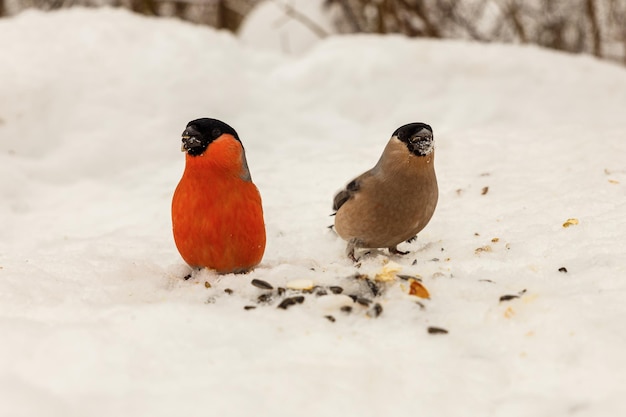In this photograph, framed in a wide vertical rectangle, two birds are captured amidst a serene snowy landscape. Both birds appear to be of the same species but exhibit different coloration. The bird on the left features a striking black head and back, with a vibrant deep dark orange chest and neck. Its black legs are obscured by the snow as it forages. The bird on the right shares the black head and back but has a brown chest and neck. Unlike its companion, the tops of its black legs are slightly visible above the snow. Both birds have their wings and feathers pulled up behind them and their black pointed beaks are dusted with tiny flecks of snow, evidence of their activity. Scattered around them are multiple black, brown, and tan-colored seeds, which they seem to be pecking at. The snowy ground curves gently upwards towards the back of the photo, where thin, leafless branches of trees or bushes are faintly visible, adding a touch of texture to the tranquil scene.